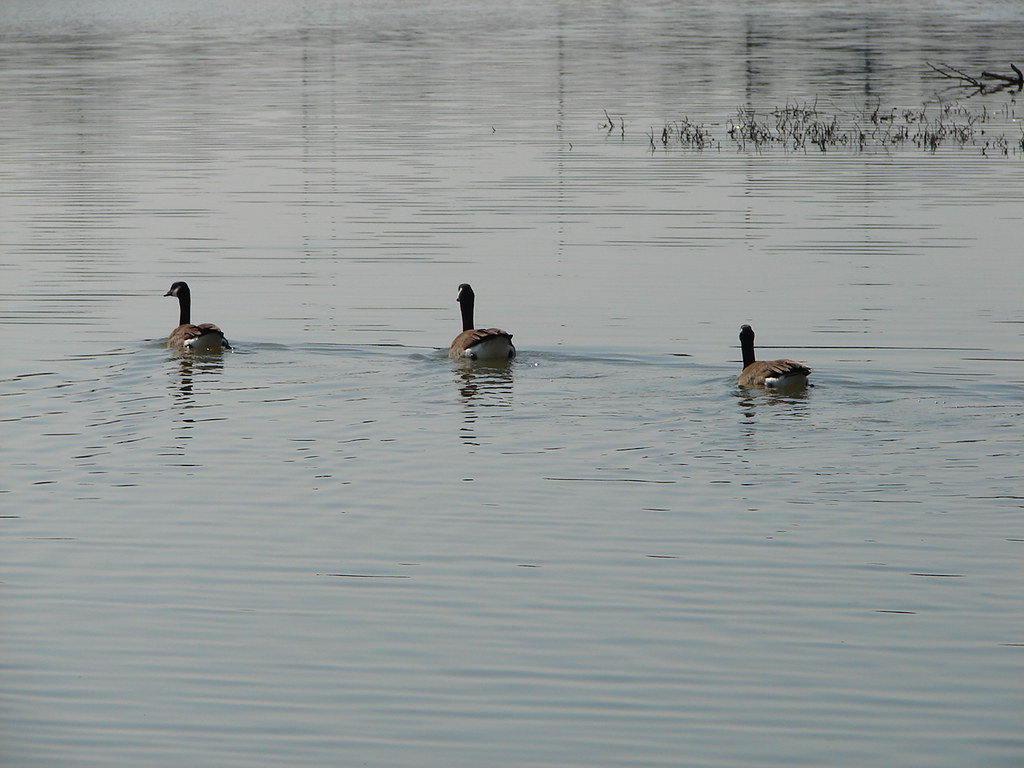In this serene image, three Canadian geese swim gracefully in a calm body of water, their wakes the only disruption on the otherwise smooth surface. The water reflects the surrounding trees, adding a touch of tranquility. The geese, identifiable by their distinctive brown bodies, white facial markings, and long black necks, are all swimming away from the camera. The goose on the left is glancing to its side, while the other two look straight ahead. In the upper right corner of the image, a few blades of grass and the tips of bare branches protrude through the water, hinting at the shallow depth in that area. The lighting suggests it may be early morning, late afternoon, or perhaps an overcast day, shrouding the scene in a gentle, diffused light.